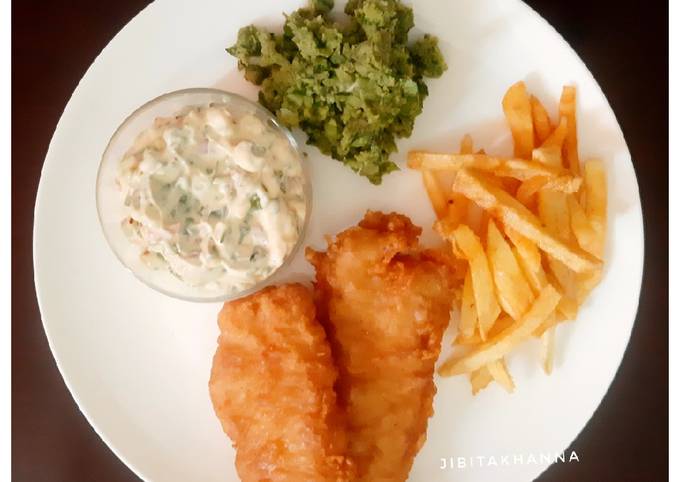This detailed close-up photograph, taken from above, features a white dinner plate on a dark, chocolate brown table. The plate contains four distinct elements. At the bottom of the plate lie two golden-brown, crispy fish fillets, with the one on the right displaying more vibrant red and orange accents compared to the one on the left. On the right side, there is a small hand-sized portion of orangish-yellow French fries. At the top of the plate, a serving of steamed, chopped broccoli is visibly green and vibrant. On the left-hand side, a small clear glass bowl contains a white tartar sauce with flecks of green, orange, and yellow mixed in. Adding to the presentation, there is text over the plate that reads, "J-I-B-I-T-A-K-H-A-N-N-A." The primary colors in the image are the golden hues of the fish fillets and fries, the white of the plate and sauce, and the green of the broccoli, all set against the dark table background.